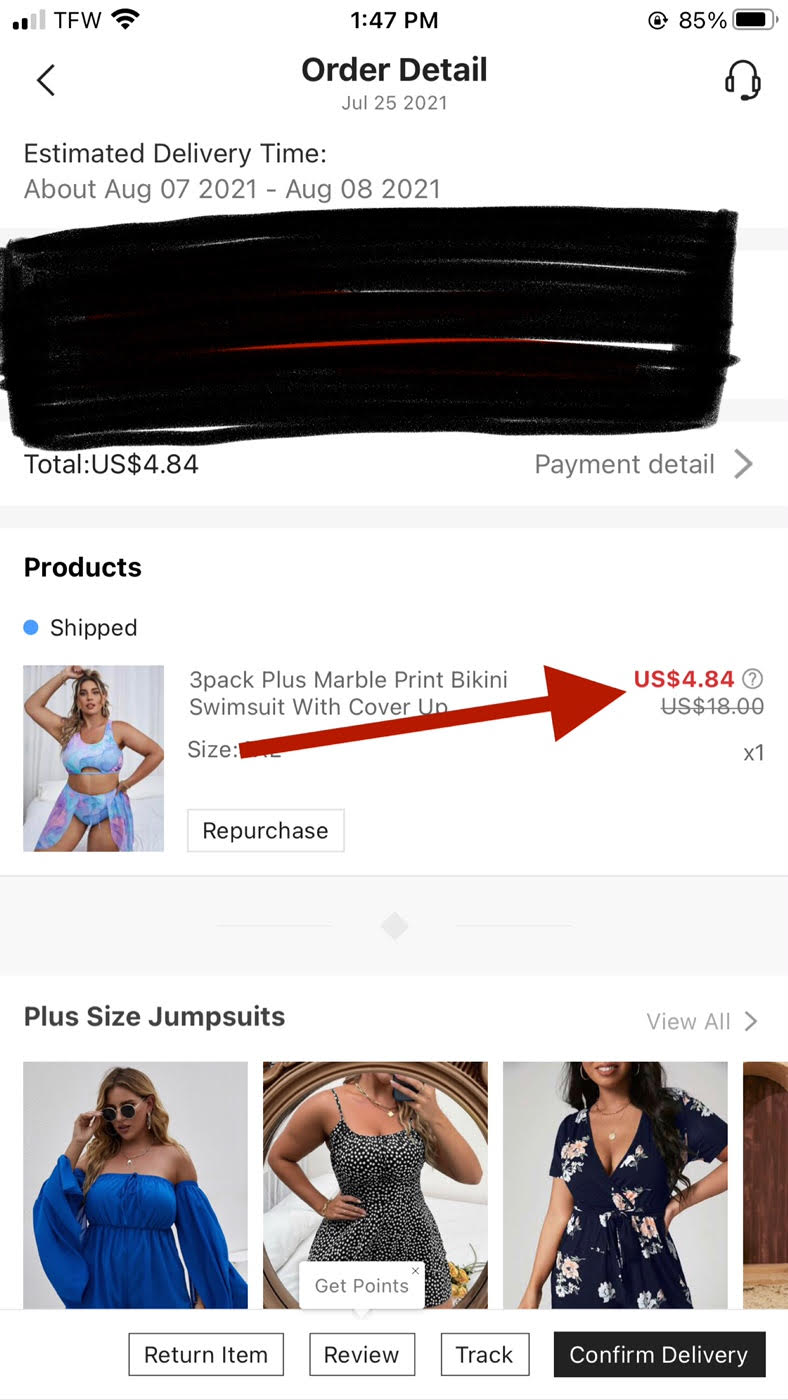The image appears to be a screenshot of a phone display, capturing a digital order detail page. At the top of the screenshot, "Order Detail" is prominently displayed in bold, black text. Just below this, there is a section labeled "Estimated Time Delivery" with the information underneath obscured by black marker scribbles.

Following this obscured section, there are three separate rectangles. The first rectangle indicates an estimated delivery time frame of "August 7, 2021 - August 8, 2021," followed by more black marker obfuscations. Below the blacked-out section is the total amount, listed as "$4.84."

Further down is another section labeled "Payment Detail," accompanied by an arrow prompting the viewer to click to the right. Underneath this is a rectangle labeled "Products," featuring a small blue dot labeled "Shipped." Next to this is a thumbnail image of a woman wearing lingerie or swimwear, and the description reads "Three-pack Plus Marble Print Bikini Swimsuit with Cover-up." The price "$4.84" is prominently displayed in red next to a bold red arrow also pointing to this amount. Beside it, there is a "Repurchase" button.

At the bottom of the screenshot, there is mention of "Plus Size Jumpsuits" accompanied by thumbnail images of three different styles: a bright blue jumpsuit, a black and white animal print jumpsuit, and a black flowery jumpsuit. Beneath these images are four buttons labeled "Return Item," "Review," "Track," and "Confirm Delivery," offering various options for order management.